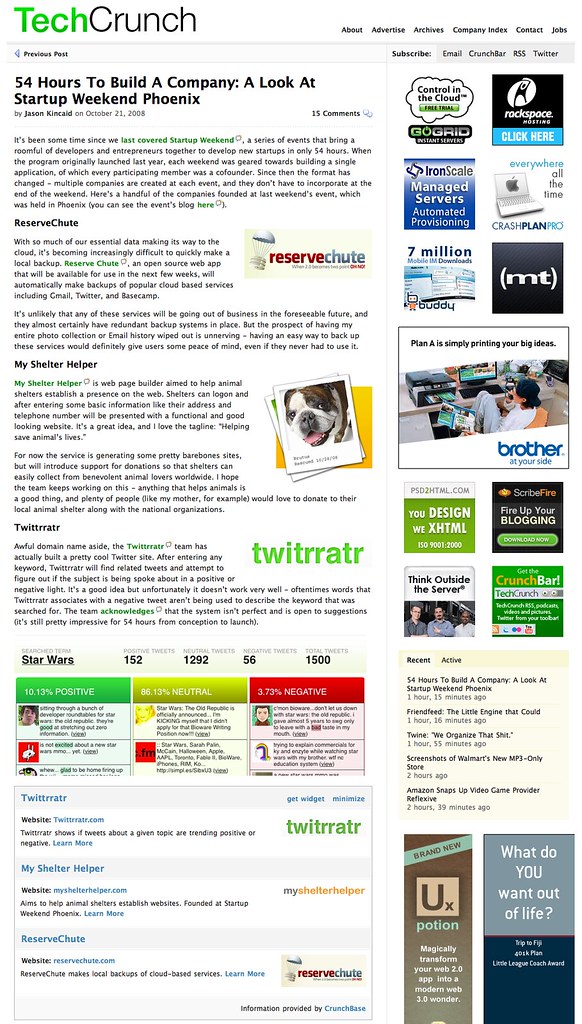This is a screenshot of a webpage from TechCrunch, identified by its distinctive green and black logo at the top left. 'Tech' is written in green with a capital T, followed by 'Crunch' in black with a capital C, forming the conjoined name 'TechCrunch.' Surrounding the logo are small black hyperlinks on the right side, leading to subcategories such as About, Advertise, Archives, Company Index, and Jobs. These are delineated by a thin gray line beneath them.

Directly below is a rectangular search box, with a series of clickable buttons including Subscribe, Email, Church Bar, RSS, and Twitter, each labeled in small black uppercase text. A gray line further separates this upper section from the main body of the page, which predominantly features a white background.

The main content includes a prominent headline in large black letters: "54 hours to build a company: a look at startup weekend Phoenix." This article is authored by Jason [last name unclear], dated October 21, 2008. There are 11 comments noted to the right of the heading. The content further breaks down into five key sections, each beginning with bold headers. The first is "Reserve Shoot," accompanied by an image of a branded rectangular item with 'Reserve' in red and 'Shoot' in blue. Following the text for this section are additional sections labeled 'My Shelter Helper' and 'Shelter Helper' (the latter in green text), interspersed with multiple paragraphs separated by large black headings.

To the right of these paragraphs, there are stacked Polaroid-like images, including one of a bulldog under the "My Shelter Helper" heading.

Towards the bottom of the page, another gray line divides sections of information and images. Highlights include a green block labeled "Star Wars," a gold section with a mix of paragraphs and gray squares, a red section with paragraphs mixed with white-lettered headings, and a grayed-out block featuring blue headings. 

On the far right side, the page displays vertical rows of six small advertising blocks, a large advertisement for Brother—featuring a man at a computer with the slogan "At Your Side" in blue—and additional advertising blocks interspersed with paragraphs. The final section contains light tan and gray-blue blocks with text.

Overall, this screenshot captures the structure and detailed layout of a TechCrunch webpage, featuring various articles, advertisements, and navigation options.